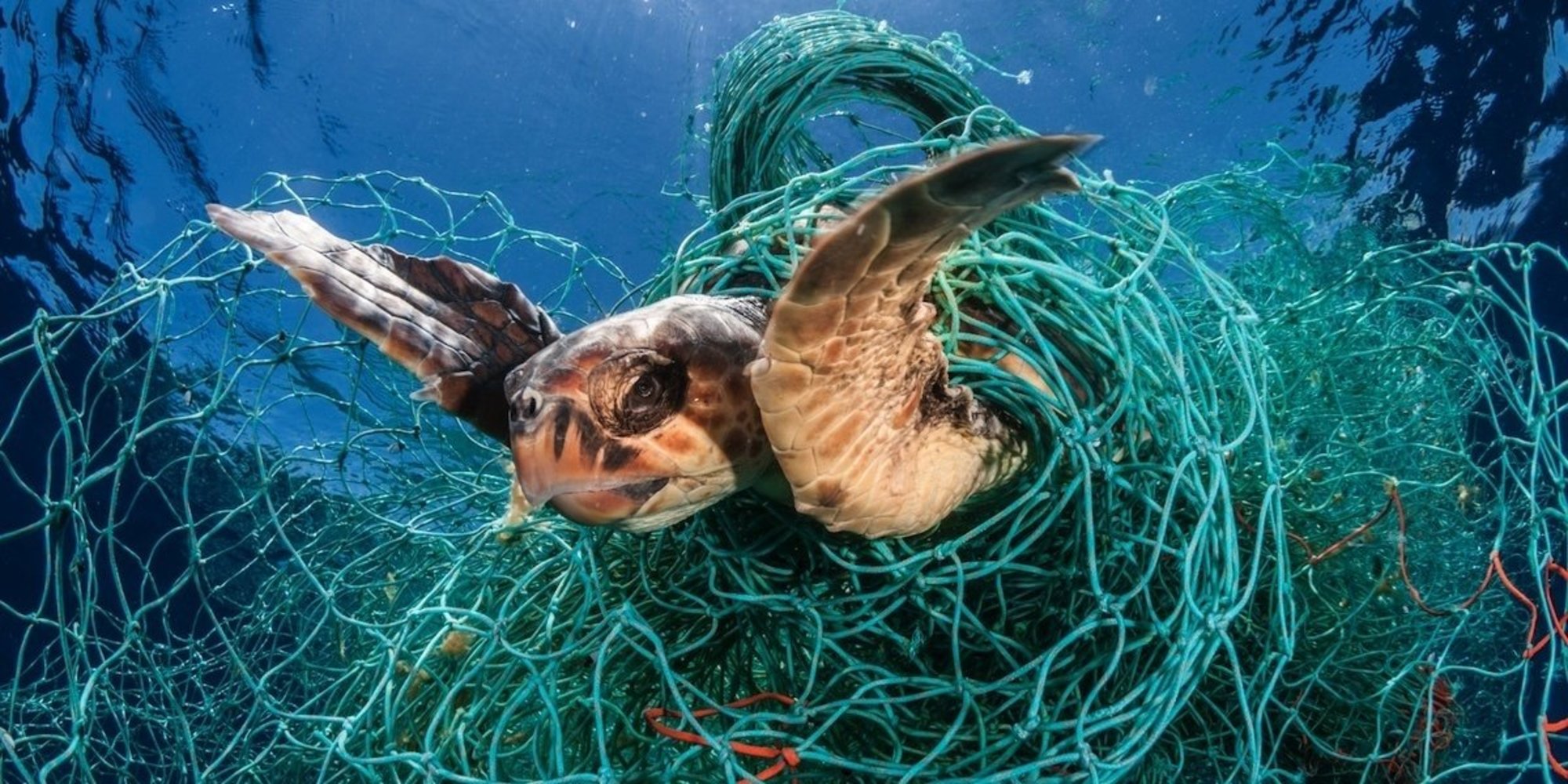In this detailed underwater photograph, a sea turtle is depicted ensnared in a tangled mass of plastic netting, primarily turquoise green. The turtle, trapped and unable to move freely, has its dark brown, dinosaur-patterned head and flippers protruding while the rest of its body is obscured by the net. The brownish head features dark, somber eyes and a closed beak. The sea turtle is centered in the frame, engulfed by the netting, with the blue ocean and shimmering surface of the water visible above, indicating its proximity to the surface. Various colors such as reddish, tan beige, and orange can be seen interspersed in the scene, adding to the stark contrast and highlighting the distressing circumstance of the turtle. The overall clarity of the photograph vividly captures the plight of the ensnared turtle, evoking a deep sense of urgency and sorrow.